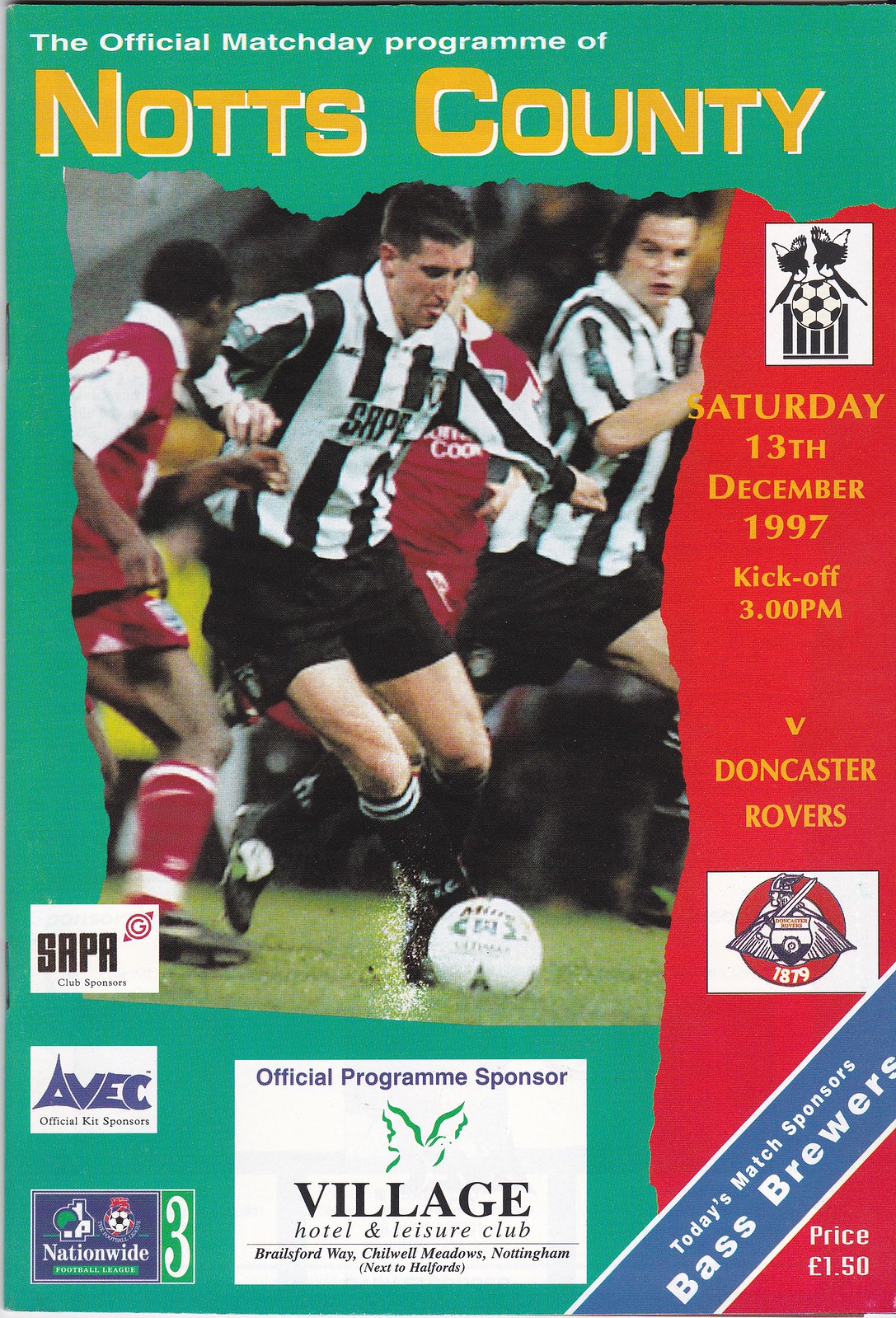The image is the cover of an official match day program for a soccer game, predominantly featuring a green background with a red section on the right. At the top, white text reads "Official Match Day Program," followed by large yellow letters spelling out "Knott's County." In the center, there's an action photograph depicting a soccer match: one player in black and white striped jersey and black shorts, with knee-high socks, is dribbling the ball, while two players in red and white jerseys are in pursuit. The scene appears to be in motion, possibly during rainy or muddy conditions as water kicks up from the field.

On the right side of the cover, beneath a logo of two birds perched on a soccer ball, yellow text states the match details: "Saturday, 13th December 1997, kickoff 3 p.m. vs Doncaster Rovers." Below this, the Doncaster Rovers' logo is depicted, featuring a man with a sword and a Viking helmet over a shield with "1879" written on it. 

At the bottom right, a blue stripe contains white text: "Today's Match Sponsors Bass Brewers." The price of the program, £1.50, is also displayed in this section. The left side of the cover showcases three rectangles with advertisements for different sponsors: SAPA in black letters on a white background, AVEC in blue letters on a white background, and Nationwide accompanied by a logo of a house, a tree, and the number three on a green background. The largest ad at the bottom center promotes Village Hotel and Leisure Club, highlighting its location at Brailsford Way, Chilwell Meadows, Nottingham next to Halfords.